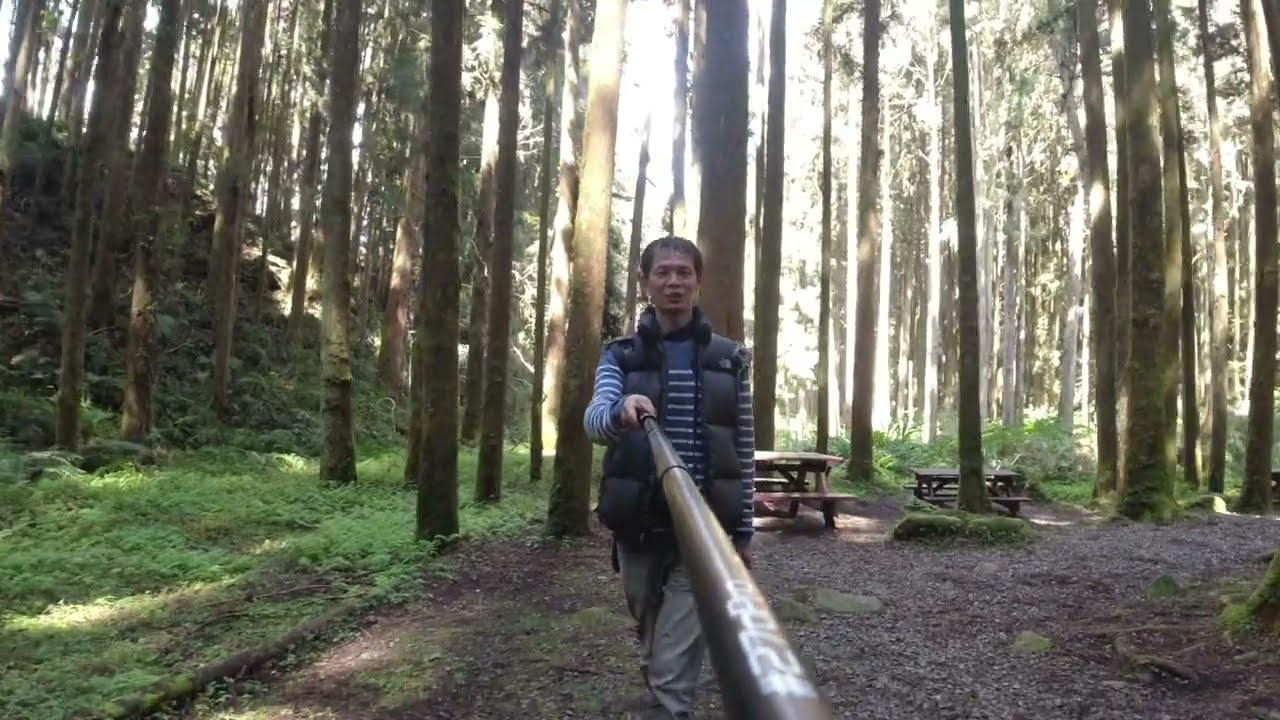In this vibrant outdoor photograph set in a forested area, a man of Asian descent stands at the center, holding a long selfie stick extended towards the viewer. He has short, dark hair and a medium build, and is dressed in a long-sleeved blue shirt adorned with thin white horizontal stripes, topped with a black puffy vest, and beige pants. The clarity of the image is exceptionally high, with bright daylight illuminating the scene, revealing intricate detail. The forest backdrop features towering, old trees, lush green grass, and assorted vegetation. A gravel path runs beneath the man's feet, and scattered picnic tables and rocks are visible further back, hinting at a day-use or campground area. No other people or text are present in this sharp, well-lit, landscape-oriented photograph that captures a moment of serene realism.